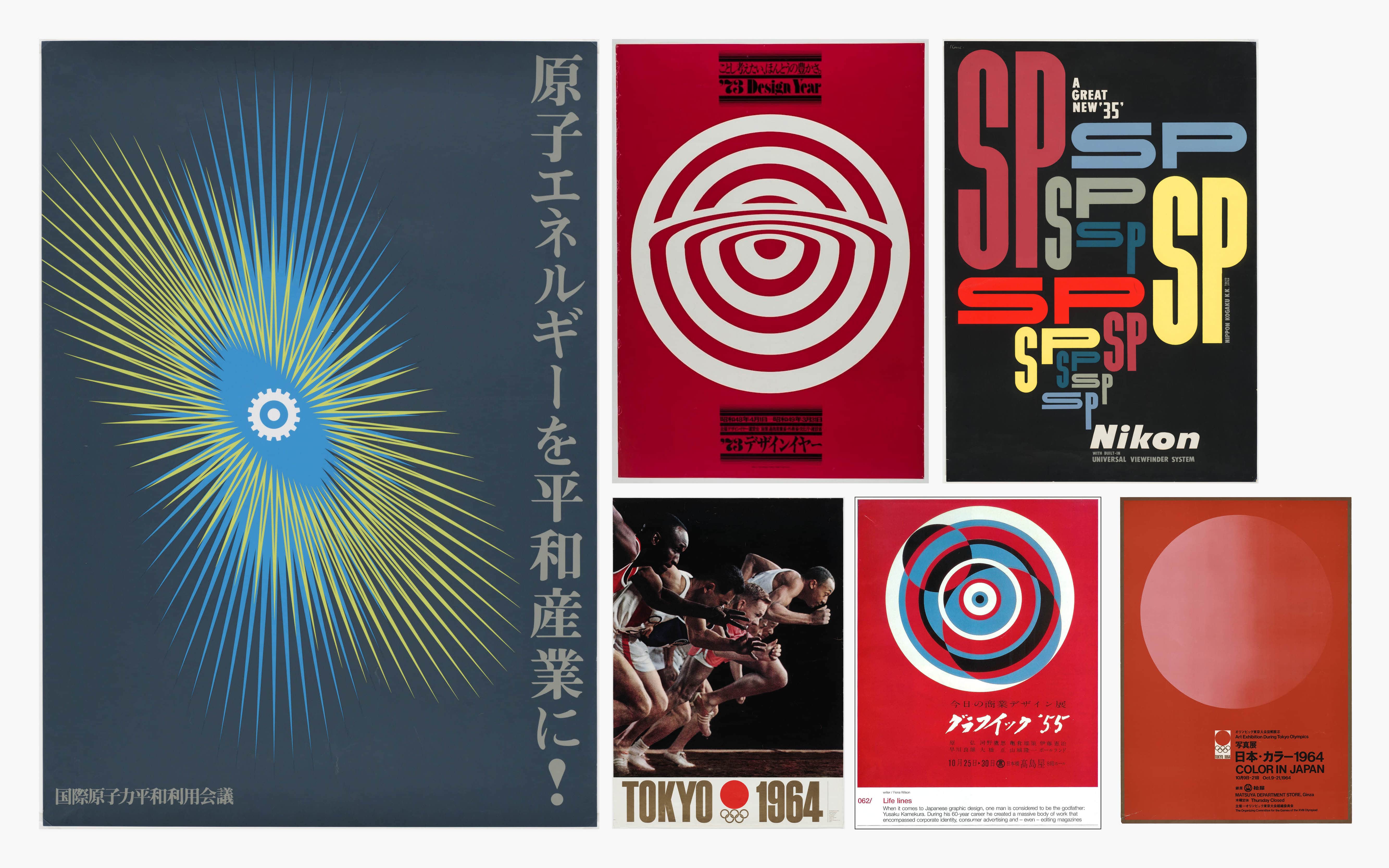The image is a vibrant collection of six Japanese posters, each showcasing unique designs and themes. Dominating the left side is the largest poster, featuring an oval shape with gold lines radiating outward against a dark blue background, with numerous Japanese characters, including the katakana for "Energy." To the right, the top row comprises two smaller posters. One of these is for the Tokyo 1964 Olympics, depicting runners on a track, while the other boasts a Nikon advertisement with a black background and colorful letters spelling "SP" in various fonts. The bottom row contains three posters, all characterized by red backgrounds. One exhibits a coral-colored globe, another features a trippy variation of a red and white bullseye reminiscent of the Target logo, and the final poster displays a complex pattern of red, blue, and white concentric circles. Each design is distinct, yet they all reflect a shared Japanese aesthetic.